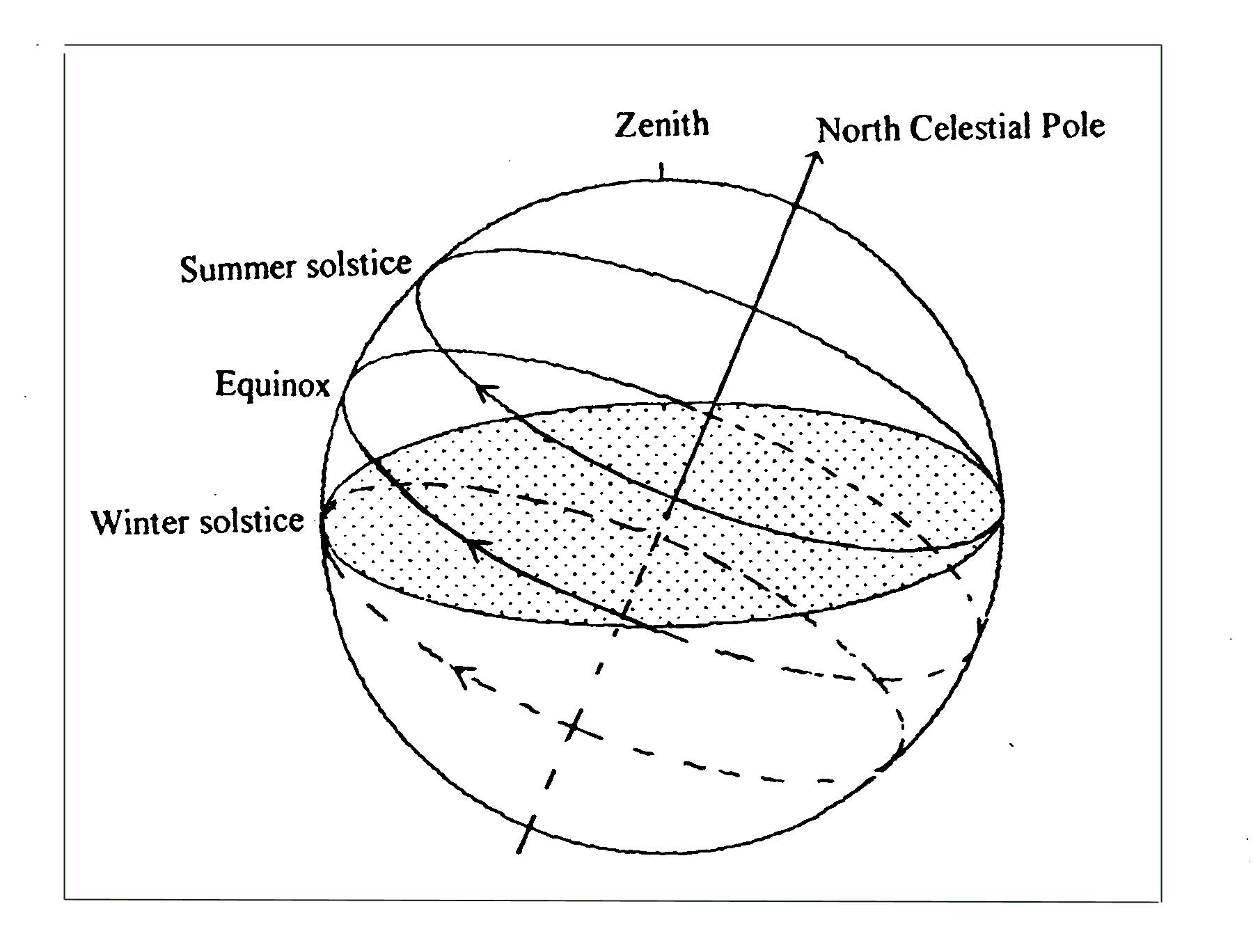This black and white scientific diagram illustrates the Earth's axial tilt and its position during the key points of the year: the Summer Solstice, Equinox, and Winter Solstice. Central to the image is the Earth, depicted as a sphere without any geographic features, emphasizing its geometric and celestial orientations. An arrow runs diagonally from the south to the north, clearly marking the North Celestial Pole at the top and its corresponding Zenith. Inside the sphere, a dotted line represents the equator, showing its varying tilt during different times of the year. The Summer Solstice, Equinox, and Winter Solstice are indicated with arrows and labels, depicting their relative positions and the Earth's tilt during each respective period. This detailed, labeled line drawing serves as a precise educational tool for understanding the Earth's axial orientation and seasonal changes.